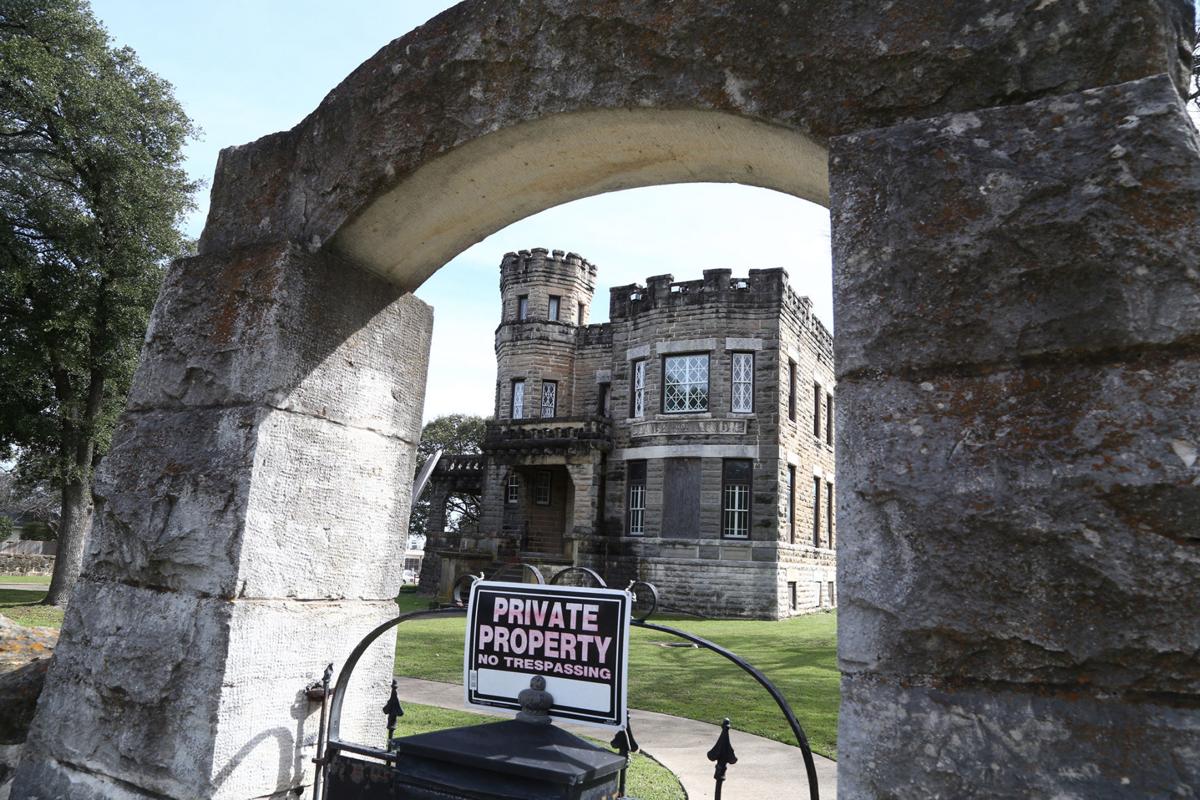This full-color, square photograph was taken outdoors on a partly sunny day. Dominating the scene is an old, fancy gray brick building designed to resemble a castle, though it's more of a two-story house. Notably, it features a traditional round turret on the left side, giving it a three-story tower appearance. The right side of the building is flat-roofed, and the front has a long, covered porch. There are several windows with grid patterns inside them. The entryway to this property has a picturesque stone archway with large square stones, supporting a black metal gate with a "Private Property, No Trespassing" sign. Lush, well-maintained grass surrounds the area, with a large, leafy, dark green tree to the left. The sky above is a light blue, enhancing the castle-like yet intimate charm of the scene.